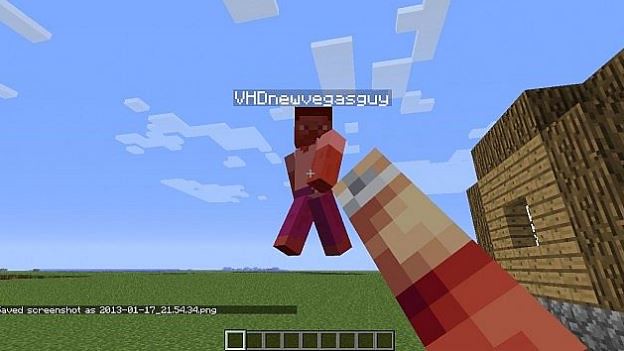This image showcases a scene from a video game bearing a strong resemblance to Minecraft. The landscape is a grassy green surface, indicative of classic block-style terrain. To the right, a structure made of brown wooden blocks is visible, featuring a small window cut out, allowing light to seep through. The base of the structure is constructed from grey stone blocks, adding a sturdy foundation.

Central to the foreground, a rod or stick composed of small, multicolored blocks extends from the bottom towards the top of the frame. Its colors—beige, brown, red, orange, and possibly pink—create a textured, cube-like appearance.

Behind this rod stands a small character. The figure is dressed in red pants and a pink shirt with red sleeves. The character has dark brown skin and black hair shaped into a box haircut. Their eyes and some facial features can be distinguished.

In the bottom-left corner of the image, a text box displays the filename: "screenshot as 2013-01-17-21.54.34.png." Hovering above the character, text reads "VHD, New Vegas Guy." The sky in the background is a clear blue with blocky white clouds, maintaining the game's pixelated aesthetic.